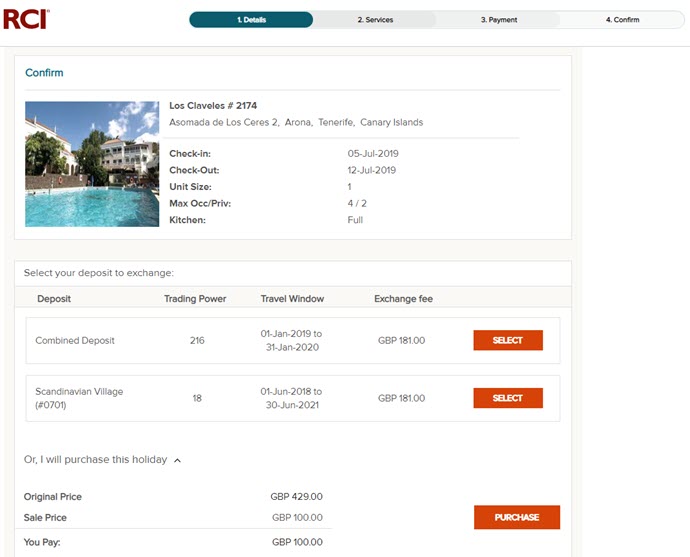RCI accommodates travelers with luxurious stays and flexible exchange opportunities, as depicted on their webpage. Prominently featured are two stunning buildings encircling a sparkling pool, flanked by verdant palm trees under a vibrant blue sky dotted with fluffy clouds. The location, identified as "Los Clavels," holds the listing number 2174 and is situated in the Canary Islands. Details beside the image indicate a check-in date of July 5, 2019, and a checkout date of July 12, 2019. The accommodations include a one-bedroom unit with a maximum occupancy of either four adults or two adults with two children, complete with a fully-equipped kitchen.

At the top of the page, users can navigate through tabs labeled "Details," "Services," "Payment," and "Confirm," offering streamlined access to essential information. In the center, options for deposit exchanges are provided, including combined deposits and trading power from locations such as the Scandinavian Village, hinting at a timeshare model where users can trade holidays for monetary value.

Prominent orange buttons on the right side simplify selection and purchase procedures. Users can clearly see their purchase options, including details on price and any available sale prices. The process culminates with a conspicuous orange "Purchase" button, ensuring a straightforward booking experience.